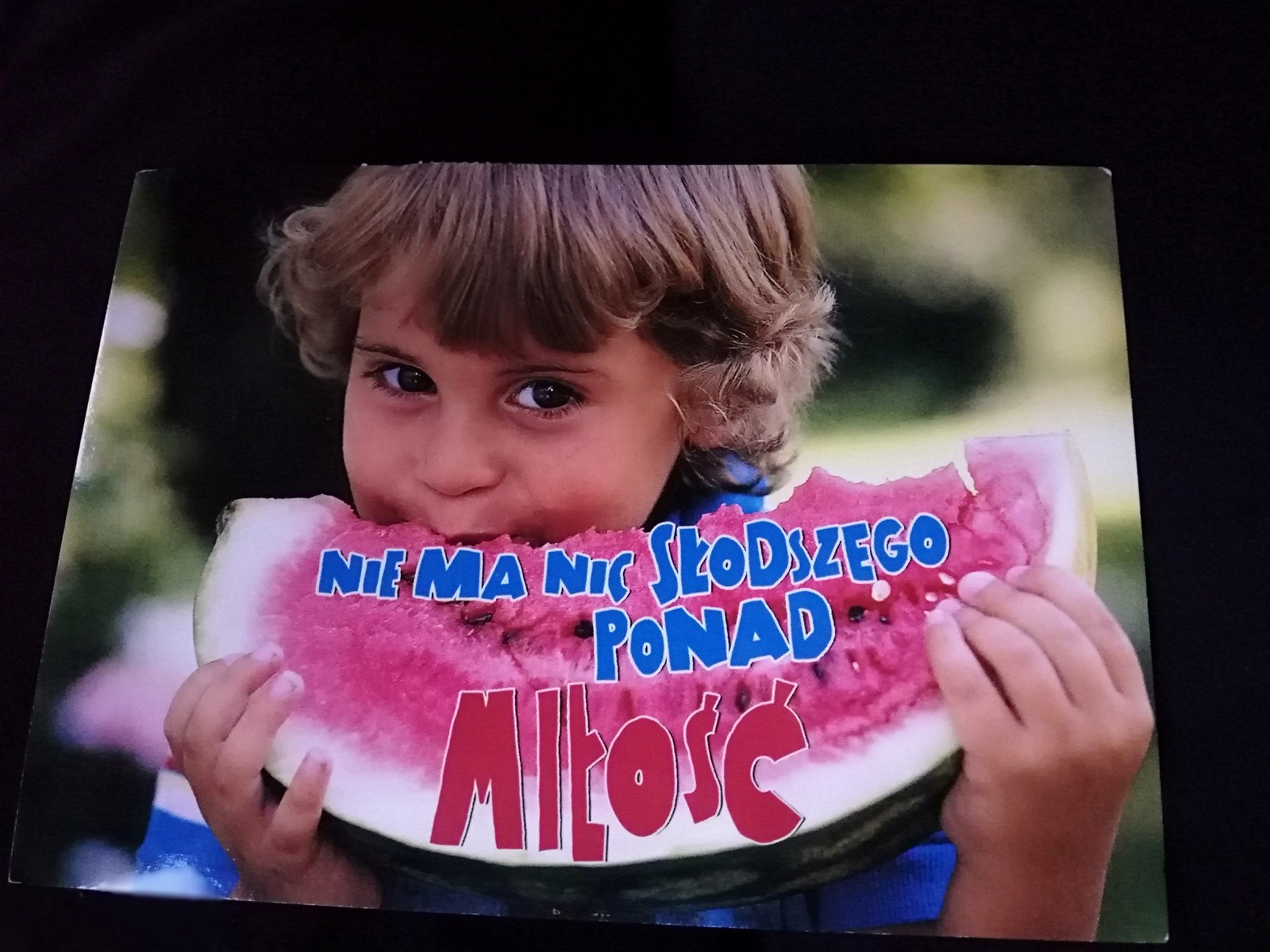The image is a color photograph with a landscape orientation, framed by a solid black border that is thicker on the top and left sides, creating an off-center tilt that gives the impression of the photograph leaning backwards. It depicts a young Caucasian boy, approximately 7 years old, with short, curly brown hair and large brown eyes. He is holding a large slice of watermelon up to his mouth with both hands, actively eating it. Across the top of the watermelon, there is blue text outlined in white that spells out a foreign phrase: "N-I-E M-A N-I-C S-K-O-D-S-Z-E G-O P-O-N-A-D." Further down on the watermelon, in large red letters with a white outline, it reads: "M-I T-O-S-C." The background appears to be a blurred, outdoor nature scene, contributing to the photographic representationalism realism style. The image is placed on what appears to be a table, enhancing its perspective and depth.